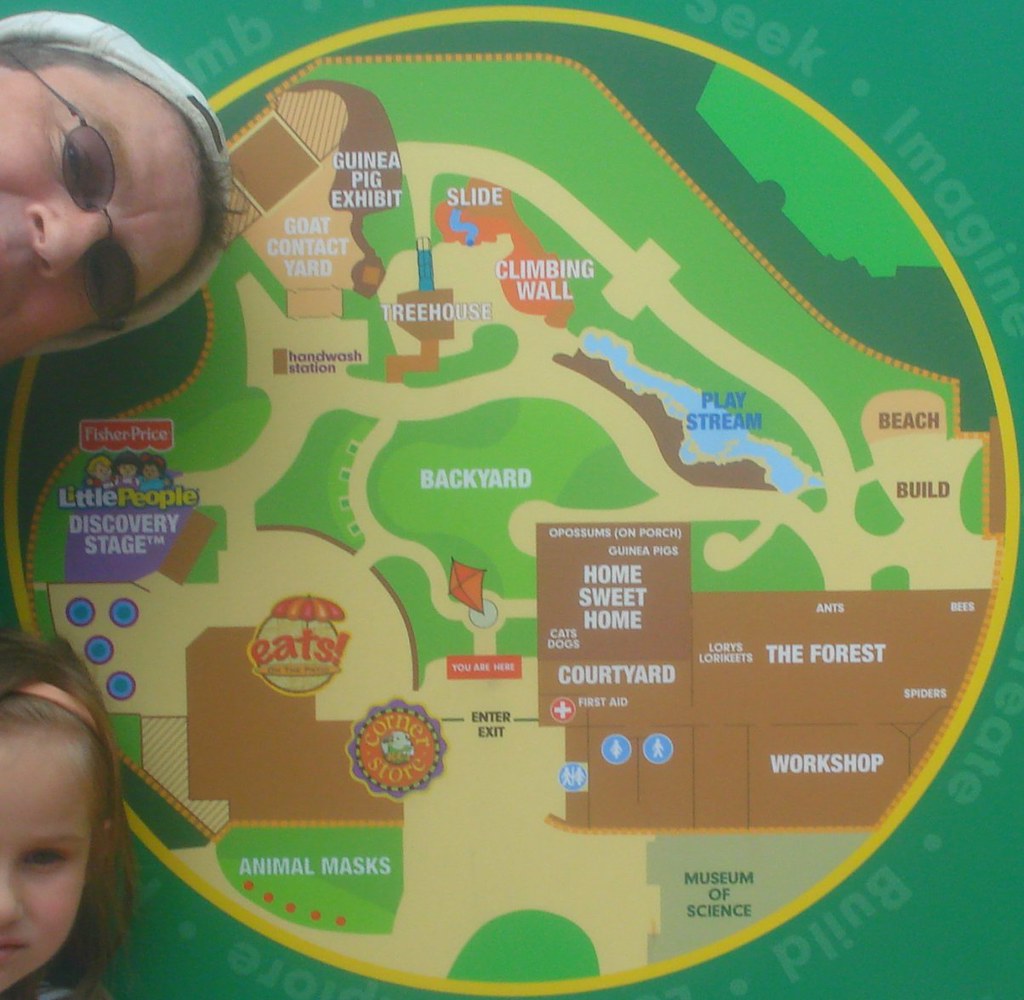The image depicts a detailed, circular map with a green background encircled by a yellow border, likely illustrating a family-oriented park or exhibit. Positioned near the top left, the partial faces of two people can be seen; one is an adult wearing a white ball cap backward and dark oval sunglasses, while the other is a young girl with blonde hair adorned with an orange ribbon. The map features various labeled areas and buildings, all marked with white text.

Starting from the bottom and moving counterclockwise, the map highlights several zones. At the very bottom, it begins with the "Museum of Science" and continues through the "Workshop," a brown building labeled "The Forest," which houses spiders, ants, lorikeets, and bees. Adjacent is the "Courtyard," followed by another brown building named "Home Sweet Home," indicating spaces for cats, dogs, possums on porch, and guinea pigs.

Continuing to the right side, at about the three o'clock position, there are sections labeled "Build" and "Beach." Near them, a water feature named "Play Stream" is shown in blue. Moving upward to the top, around the twelve o'clock position, are areas designated as the "Slide," "Climbing Wall," and "Tree House," highlighted in orange and brown. Just to the left, near the eleven o'clock mark, lies the "Guinea Pig Exhibit" in dark brown, and below it is the light brown "Goat Contact Yard." Further down, closer to nine o'clock, is the Fisher Price logo—a red rectangle with a white border and the label "Little People Discovery Stage."

Clockwise from there, at approximately the seven o'clock position, are areas marked "Eats" with an umbrella icon and "Corner Store" within the same building. Below these is a green space labeled "Animal Masks." Central to the map is a green area designated as the "Backyard," adorned with the image of a red kite and marked with a red "You Are Here" indicator near the entrance. Surrounding the "Backyard" is a variety of interactive and educational zones like “Guinea Pig Exhibit,” “Goat Contact Yard,” "Workshop," "The Forest," and "Home Sweet Home," creating a rich and diverse environment for visitors.